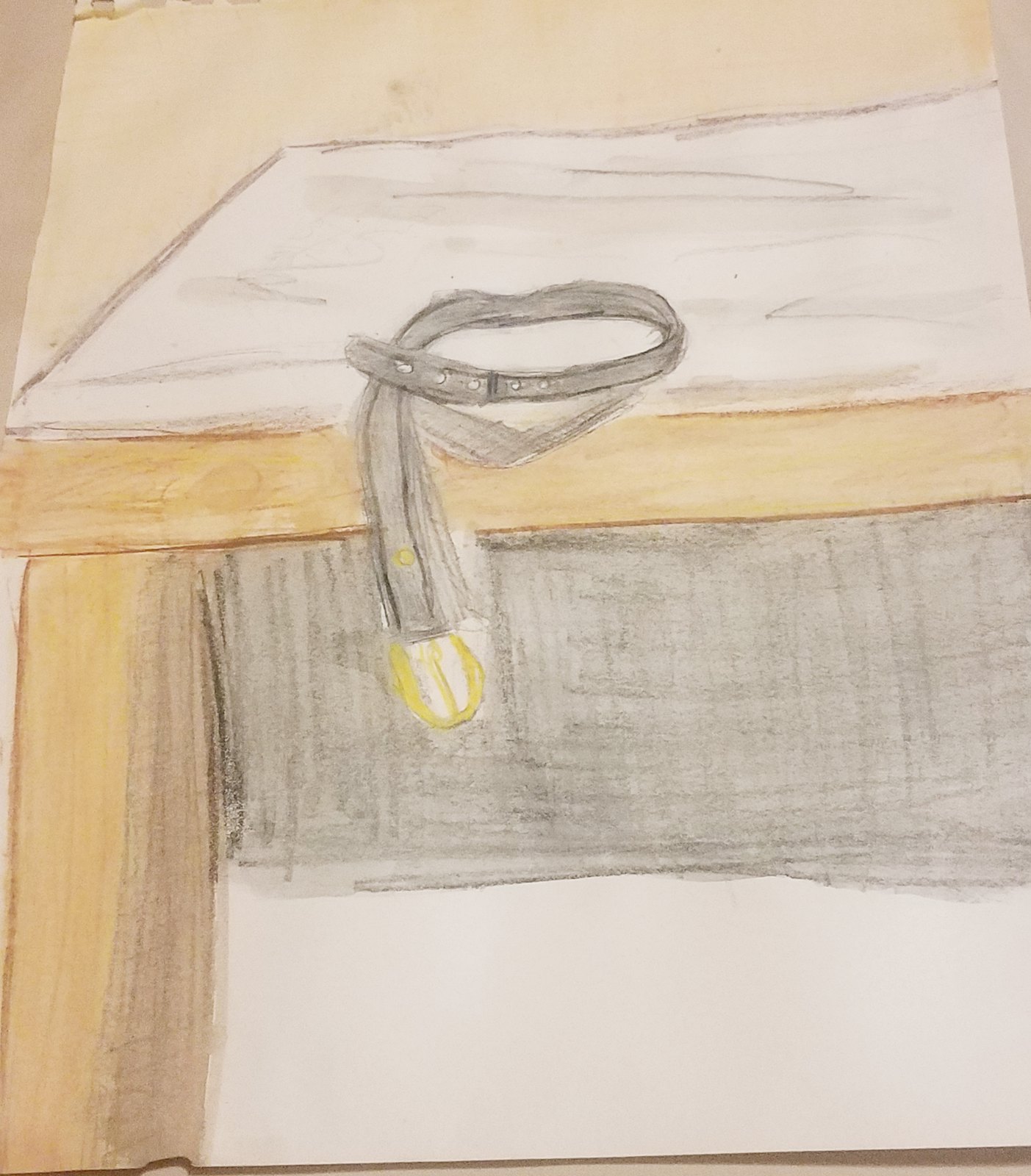The image is a detailed crayon drawing on a piece of white paper, depicting the front left leg and part of the seat of a chair. The chair leg and seat are shaded in a yellow-orange-brown color mixture, with darker shading on the leg for depth. At the bottom of the leg, there is a black base, which is lightly shaded. The chair seat features a white cushion, accented with fine black lines for dimensionality. Hanging from the chair is a black collar, resembling either a doll's or a cat's collar, with small holes and sections of darker shading where a metal clasp would connect. A gold hoop and centerpiece dangle off the collar, adding a touch of detail to the composition.

This drawing also includes aspects that make it appear like a 3D illusion of a desk. The table surface is white with light shading, bordered by a color resembling light oak wood, similar to the leg. Underneath, there's extensive black shading forming a rectangular shape, and a black belt-like object is positioned beneath, with a gold buckle prominently hanging off its end. The belt is intricately shaded in black and gray, contributing to the overall depth and realism of the drawing.